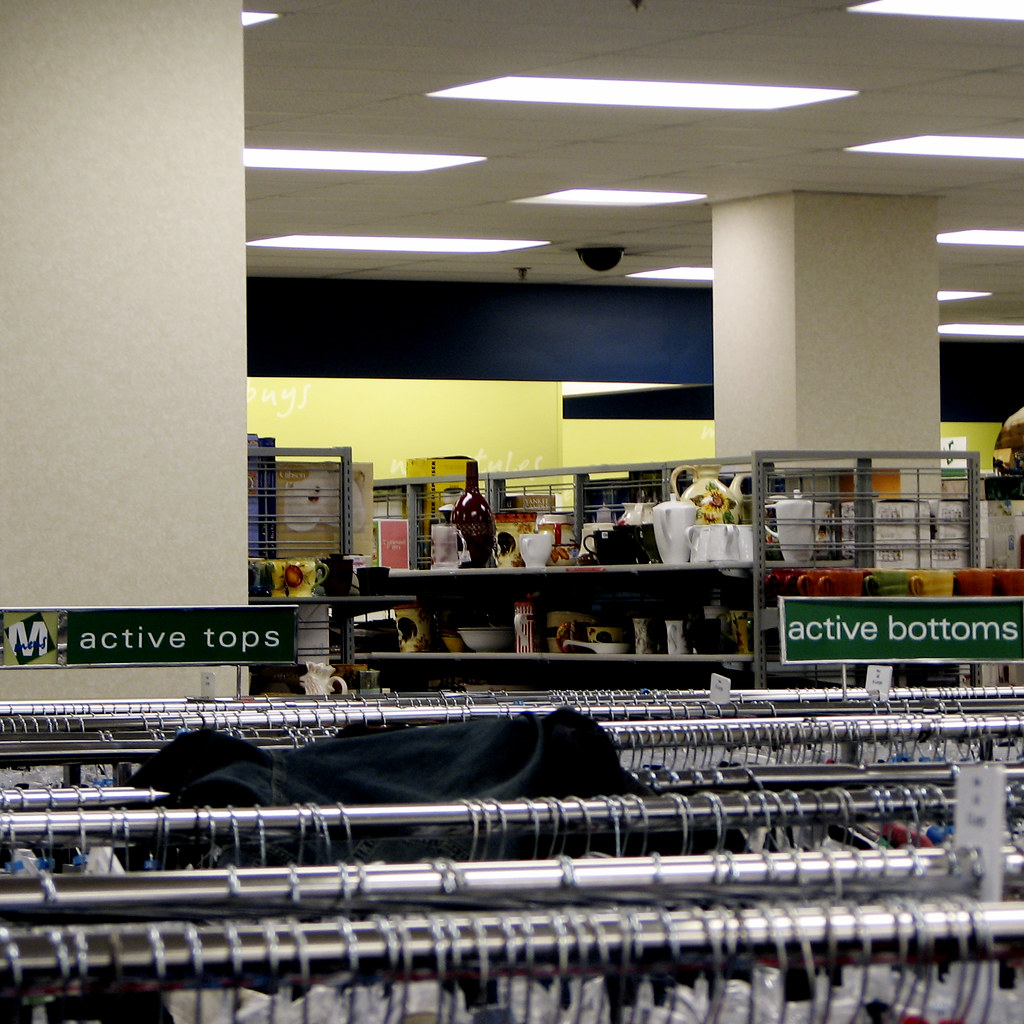This color photograph captures a detailed scene inside a large retail store, potentially a thrift store. The foreground and mid-ground feature several rows of chromatic, grey cylindrical racks populated with clothing hangers and garments, identified as men's active tops on the left and active bottoms on the right based on prominent signs with white writing. The tops of various hangers are visible, but the clothes themselves are not clearly displayed. In the background, shelves display a variety of objects typical of a thrift store, including mugs, vases, teapots, and used electronics. 

The ceiling is greyish with rectangular fluorescent and square white lights. Additionally, a black globe-shaped object, possibly a security camera, is mounted on the ceiling. Two large grey posts are present, one on the left and another further back on the right. The background wall is divided into segments: white trim at the top, a dark blue section beneath it, followed by a light yellow portion at the bottom. There is also some writing visible on the yellow portion of the wall, though it is not legible in the image. The overall ambiance and the assortment of objects and clothing strongly suggest that the setting is a thrift store.